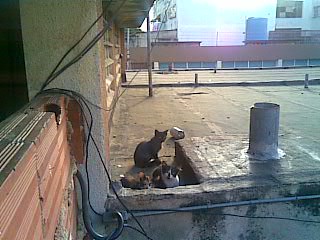This is an outdoor photograph of a rooftop scene featuring a small family of stray, feral kittens. The image is slightly grainy and low in quality. The main focal point is a group of three or four kittens, nestled at the corner of a flat cement rooftop that seems seldom accessed by people. These kittens have distinct coats: one is entirely black, another is black and white with a distinctive black nose and eye area, and the third has a brown and white coat. The black and white kitten looks directly at the camera with curiosity.

To the left of the kittens is a white wall, part of the building they're perched on, which also features a number of wires wrapped around it. This rooftop has several noteworthy details, including a cylinder or vent-like structure, a metal exhaust hose, and some pokey areas that may be vents. There’s also a rusty gate with a large metal hook and some pipes.

In the background, a red-roofed building runs horizontally, with a bit of blue sky peeking above it in the upper right. More wires and cables stretch across various parts of the scene, adding to the urban rooftop vibe. There's also the top of another building visible, showcasing windows and a bright sky overhead. Despite its small size, the photograph presents a charming glimpse into the hidden world of these young kittens exploring their elevated home.